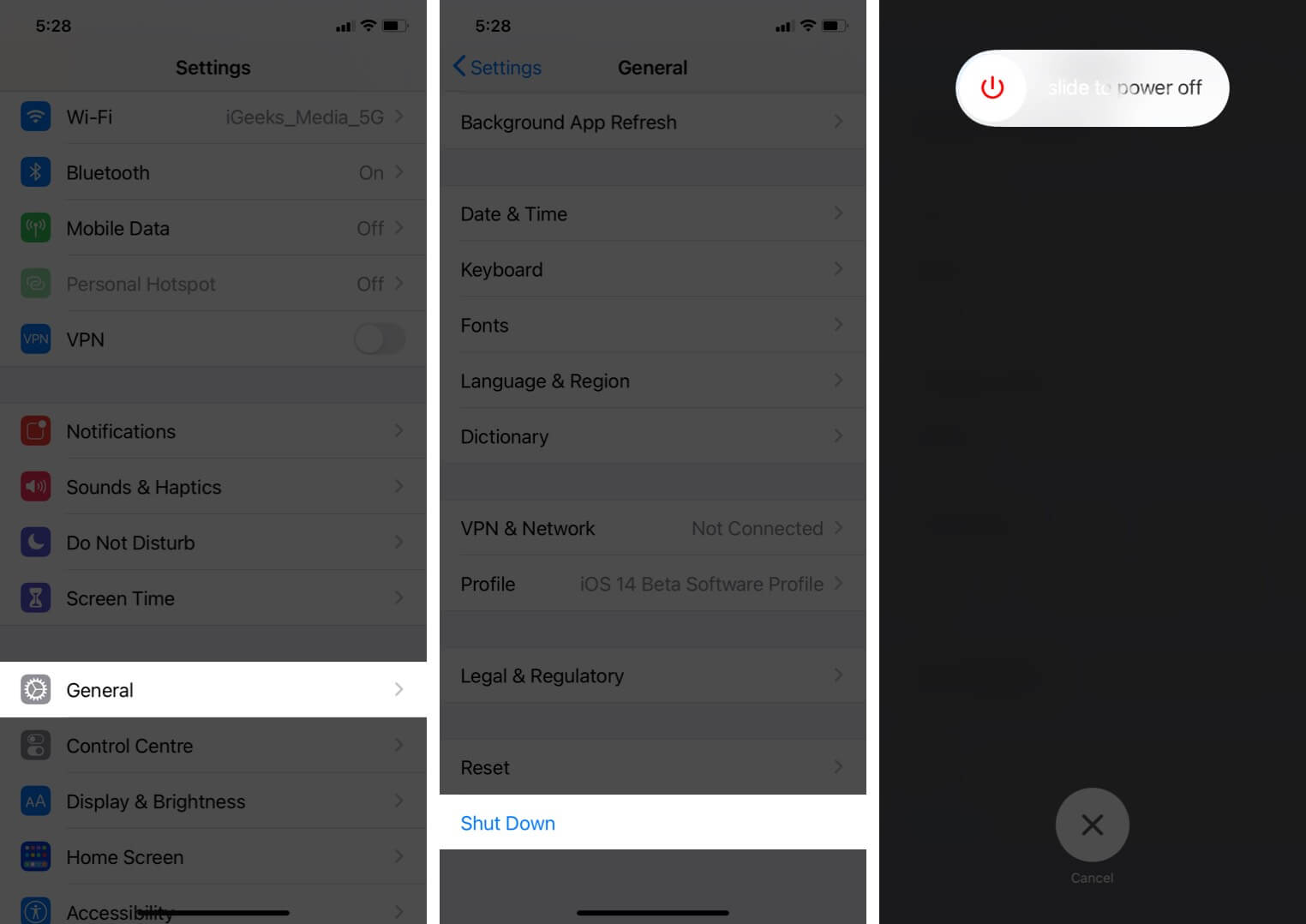Screenshot of iPhone Settings: A Detailed View

1. **Settings Menu Overview**: The top of the screen displays essential status indicators common to all iPhone pages: connection strength, battery life, and the current time. The first screenshot showcases the main "Settings" menu, highlighting several categories:
   - **Wi-Fi, Bluetooth, Mobile Data, Personal Hotspot, and VPN**: These options allow users to manage wireless connections and internet access.
   - **Notifications, Sounds, Do Not Disturb, and Screen Time**: This section helps users control alerts, sound settings, and manage interruptions and device usage.
   - **General**: Currently highlighted in this image, it includes various essential settings.
   - Below "General" are additional categories like **Control Center, Display & Brightness, and Home Screen**, offering further customization options for user interface and accessibility.

2. **General Settings Detailed View**: The second screenshot focuses on the "General" settings. Key options listed here include:
   - **Background App Refresh, Date & Time, Keyboard, Fonts, Language & Region, Dictionary**: These settings allow users to customize their language preferences, text input, and app sync options.
   - **VPN & Network, Profile, Legal & Regulatory Information**: Ensuring users can manage their network settings and understand their device's legal notices.
   - **Reset and Shut Down**: Highlighted in blue, these critical settings provide options to reset the device or power it down.

3. **Power Off Screen**: The third screenshot depicts the "Shut Down" menu, used when powering off the device. 
   - **Visual Design**: A prominent red circle with a line through the center symbolizes the power-off option.
   - **User Interaction**: By sliding this icon, users can turn off their iPhone. At the bottom, an 'X' button allows users to cancel and return to the previous screen if they choose not to power down.